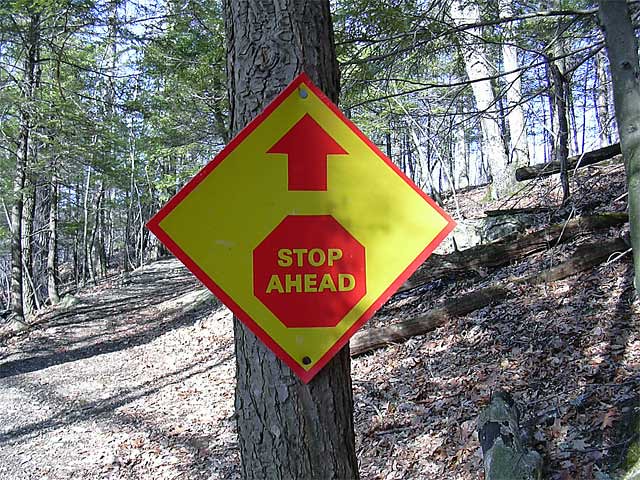The image depicts a forest scene with a clear, bright background and a steep slope descending from right to left. Dominating the foreground is a tree trunk adorned with a vivid yellow sign, outlined in a thin red rim. The sign, a rhombus positioned on its corner, features a central octagonal stop sign image accompanied by an arrow and the text "STOP AHEAD," suggesting a nearby stop junction. Surrounding this focal point, the forest comprises mostly pine and aspen trees, with their lower halves appearing barren but gradually gaining lush light green foliage halfway up. To the left of the tree, a narrow path, potentially a dirt road, winds through the forest, reinforcing the practicality of the cautionary sign in this wooded area. The scene is bathed in sunlight, highlighting the trees' evergreen characteristics against a backdrop of clear blue sky.